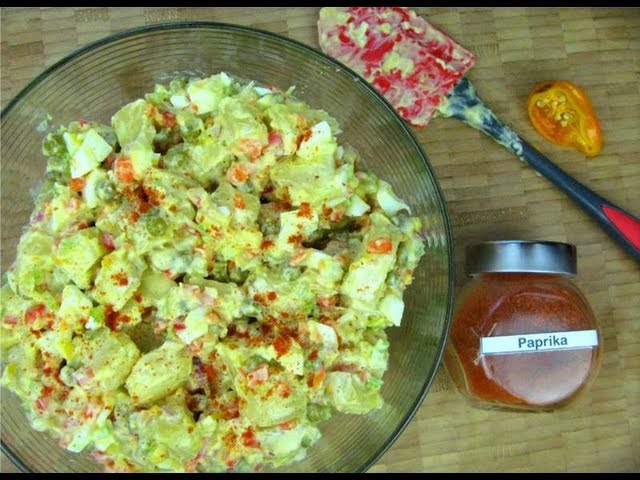This photograph, taken from a bird's-eye view, captures a vibrant, textured scene centered around a glass bowl on a wicker-style tabletop or possibly an expansive placemat. The semi-translucent bowl, featuring a black rim, contains a bright and chunky mixture resembling potato salad, accentuated with pieces of various vegetables. The salad is held together by a creamy, green dressing and sprinkled with red paprika bits, adding a colorful touch. To the right of the bowl, there's a circular spice jar with a metallic silver lid, clearly labeled "Paprika" against a white background, filled with the finely ground red spice. In the top right-hand corner, a red rubber spatula with a black handle is smeared with the salad mixture, resting near a cut orange pepper. The entire composition showcases detailed textures and colors, creating a rich, culinary still life.